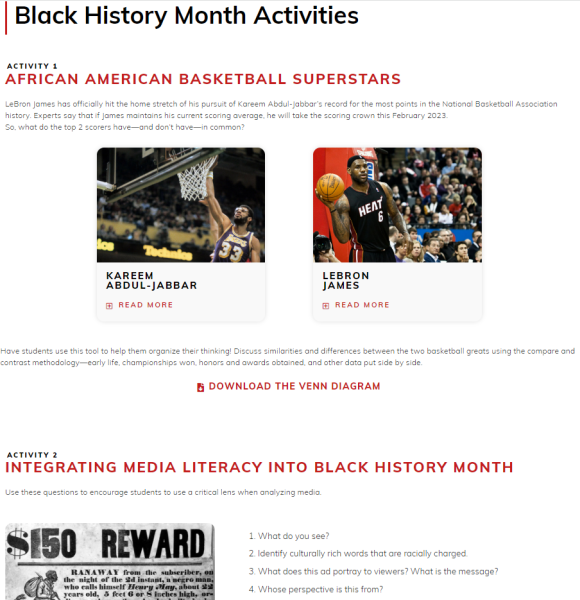The image displays a detailed printout titled "Black History Month Activities." Across the top, clear text describes an activity focused on "African American Basketball Superstars" with a spotlight on LeBron James' chase for the all-time scoring record in NBA history, currently held by Kareem Abdul-Jabbar. The text explains that experts predict James will surpass Abdul-Jabbar's record by February 2023, contingent on maintaining his scoring average. 

Highlighted below this text are two photos. To the left, a photo of Kareem Abdul-Jabbar features a clickable "Read More" option, and to the right, a photo of LeBron James similarly features a "Read More" button. Both athletes are depicted in action during a game with enthused fans visible in the background.

Further down on the page, there's a link represented in red text for downloading a Venn diagram to explore the similarities and differences between these two basketball legends. Adjacent to this link, another advertisement is displayed.

The second activity emphasizes "Integrating Media Literacy into Black History Month." The section starts with an image on the left resembling a newspaper print, albeit somewhat blurred, clearly showing a mentioning of a $150 reward. The accompanying text is divided into four distinct points, providing detailed information on the integration process.